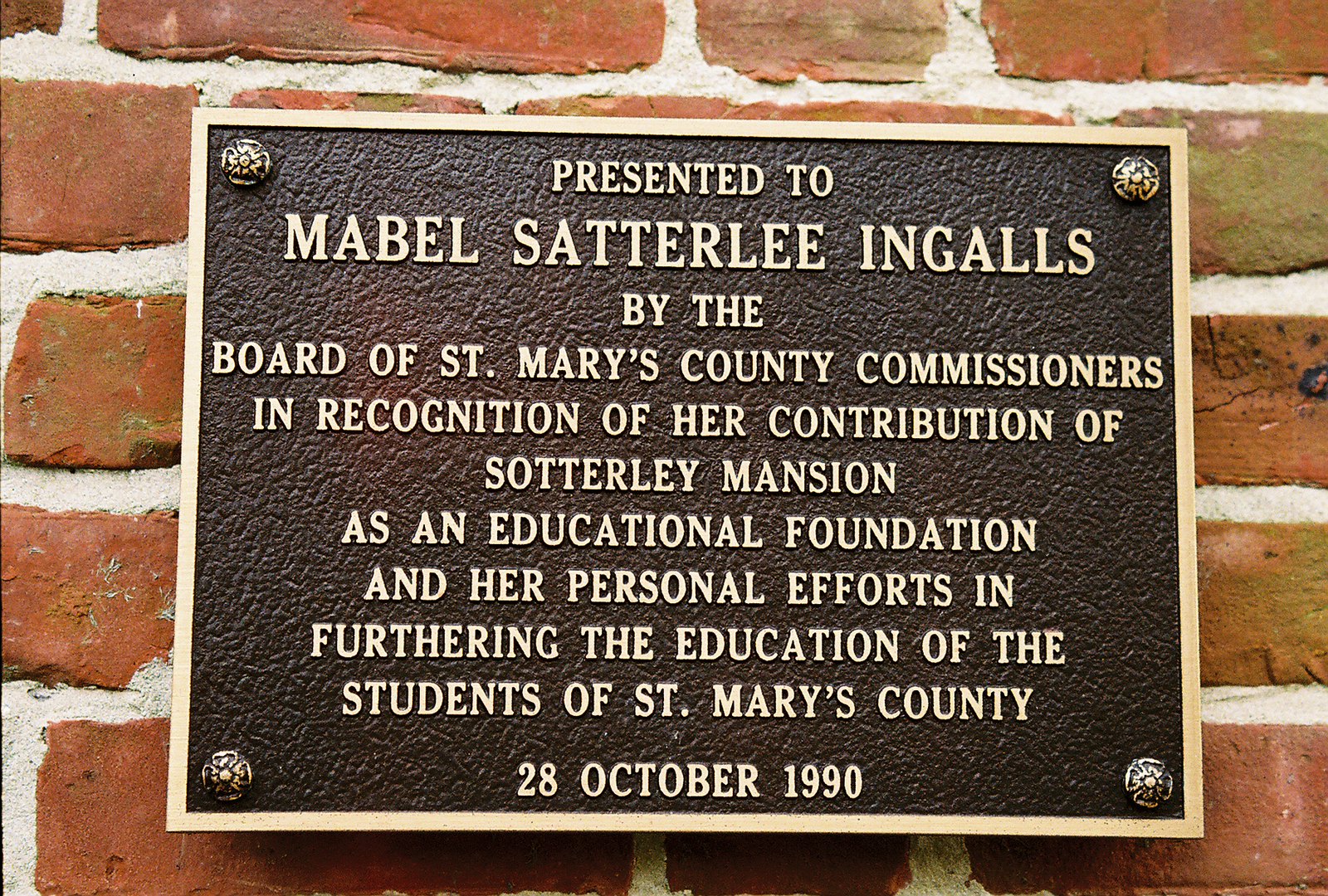The image shows a bronze plaque mounted on an old brick wall, depicting a formal recognition. This rectangular plaque has a dark background with elegant bronze or gold lettering. Each corner of the plaque is adorned with decorative bolts, contributing both to its aesthetics and its secure attachment to the wall. The text on the plaque reads:

"Presented to Abel Satterley Ingles by the Board of St. Mary's County Commissioners in recognition of her contribution of Satterley Mansion as an educational foundation and her personal efforts in furthering the education of the students of St. Mary's County. 28 October 1990."

The surrounding red bricks of the wall, with their gray mortar, create a contrasting backdrop that emphasizes the plaque's significance and historical value.